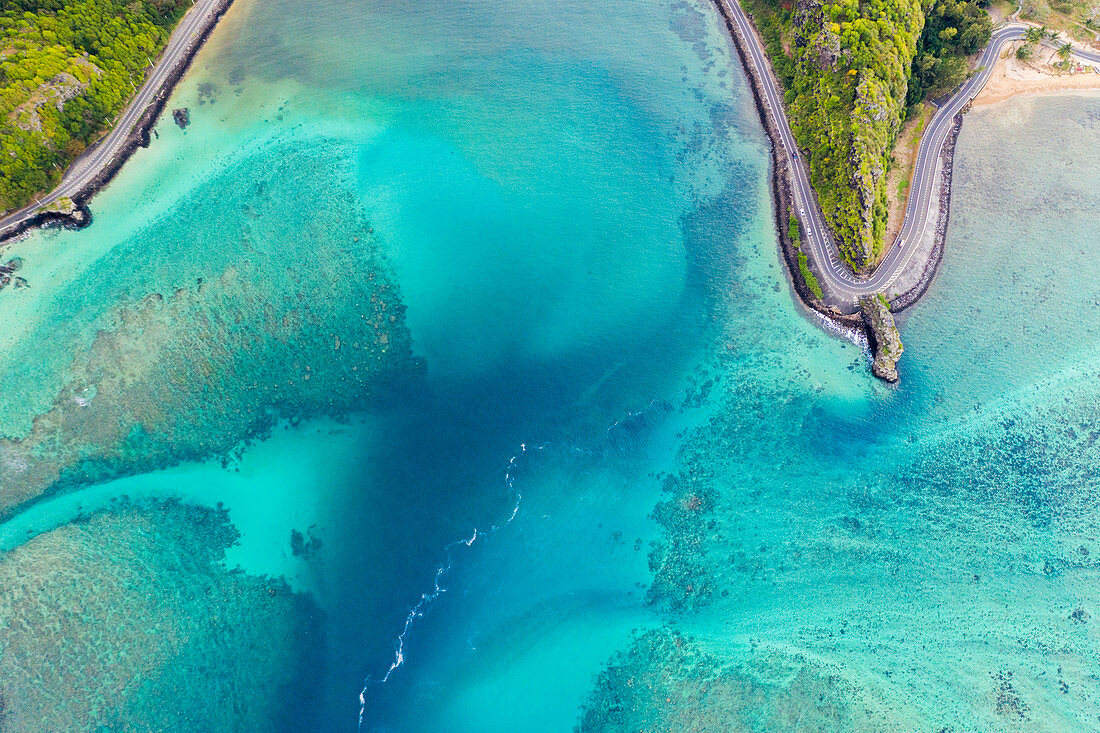The image is an aerial view, possibly AI-generated but with a photographic quality, depicting a tropical ocean scene with some land. The scene is predominantly ocean, with a myriad of blue shades, including brilliant turquoise and smudges of navy blue, indicating varying depths. Some lighter areas suggest sandy bottoms. In the top left corner, a patch of treetops in green and yellow hues can be seen, alongside a gray zigzagging road that starts here and curves up to the top right. Towards the middle-left, there's a small dock protruding into the water. The road reappears in the middle-right, winding down and then curling back up to create a U-shape, enclosing a triangular peninsula covered in vegetation similar to that in the top left, with some rocky outcrops and a tan beach area. Underneath this peninsula to the right is more clear, vibrant ocean water. This detailed portrayal, taken from high above, captures both the natural beauty and intricate landscape features of this tropical coastal area.